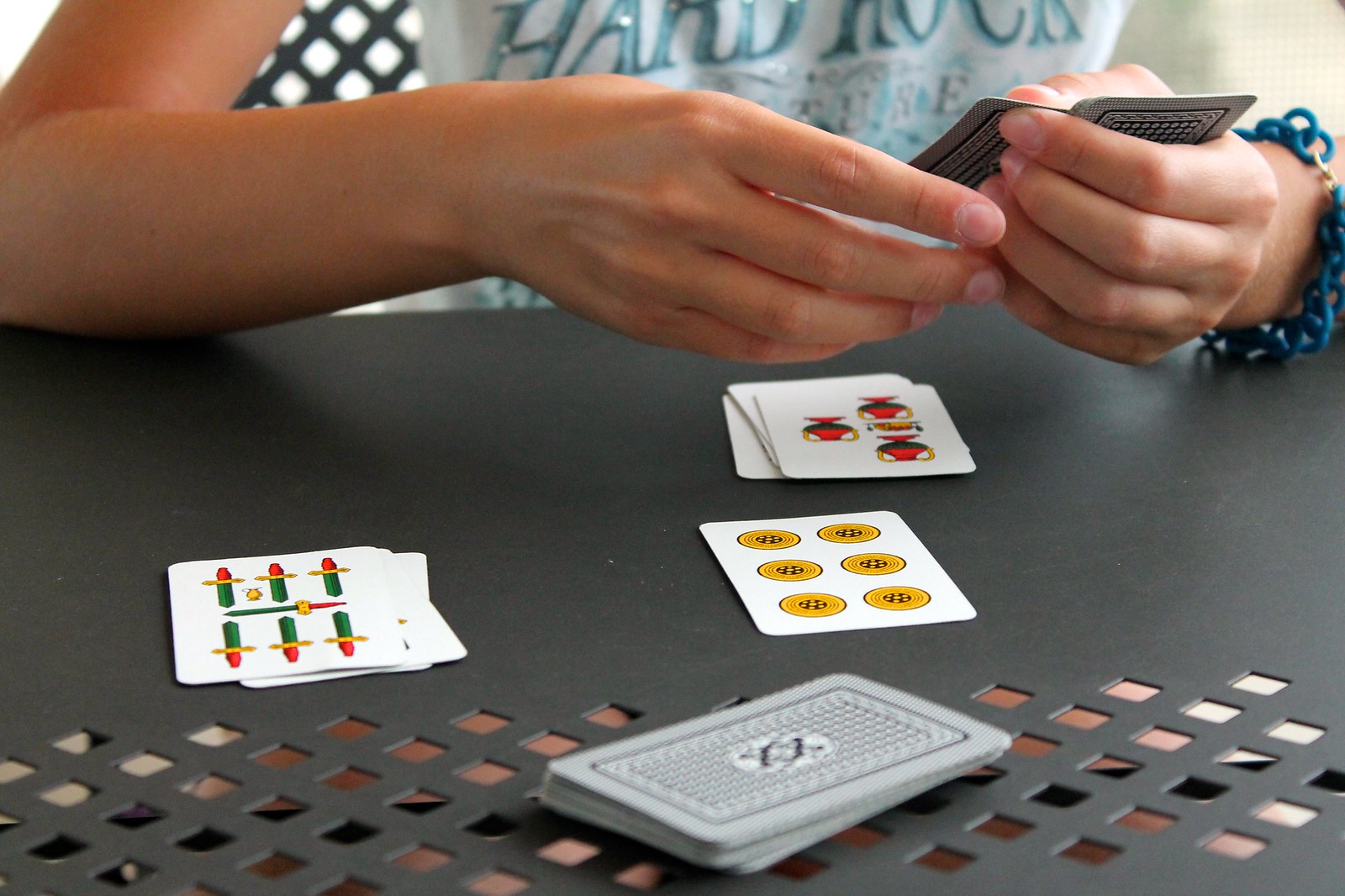A woman with tanned skin is engrossed in a card game at a wrought iron table adorned with diamond cutouts visible at the lower part of the image. She wears a distinctive blue bracelet made of curly, rubber-like material, secured by a gold clasp. Her attire includes a short-sleeved or sleeveless shirt emblazoned with a "Hard Rock" logo, revealing her bare arms and neatly trimmed short nails. In her hand, she holds two cards, their faces concealed from view. 

On the table, a central pile of cards awaits, with the topmost card featuring two X's, indicating it as the draw pile. In front of her is another pile of cards, likely her own, or perhaps her discard pile. Prominently displayed in front of her is a card marked with six yellow circles. To the right of this card lies another group of face-up cards, each depicting a green pole with yellow and red accents. The scene captures the strategic moment of the game, revealing the intricate details of the player's environment and attire.